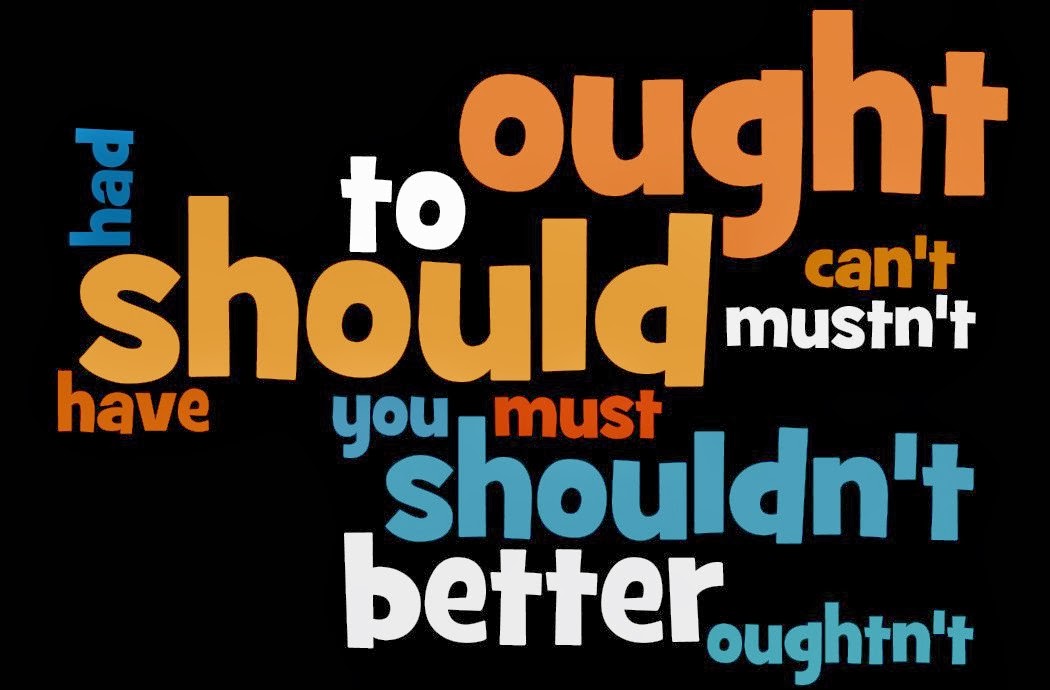This image is a piece of art or graphic design with a solid black background. It features a collection of words in various colors and sizes, all in the same font and in lowercase. The words are presented in different shades of blue, white, and orange. On the left side and turned vertically, the word "had" appears in blue. The other words, interspersed across the black canvas, include "ought," "to," "should," "can't," "mustn't," "have," "you," "must," "shouldn't," "better," and "oughtn't." The arrangement of the words does not follow a specific pattern, creating a complex interplay of text against the dark backdrop. The overall layout gives the impression that it could be a poster or a painting designed to be framed and displayed on a wall.